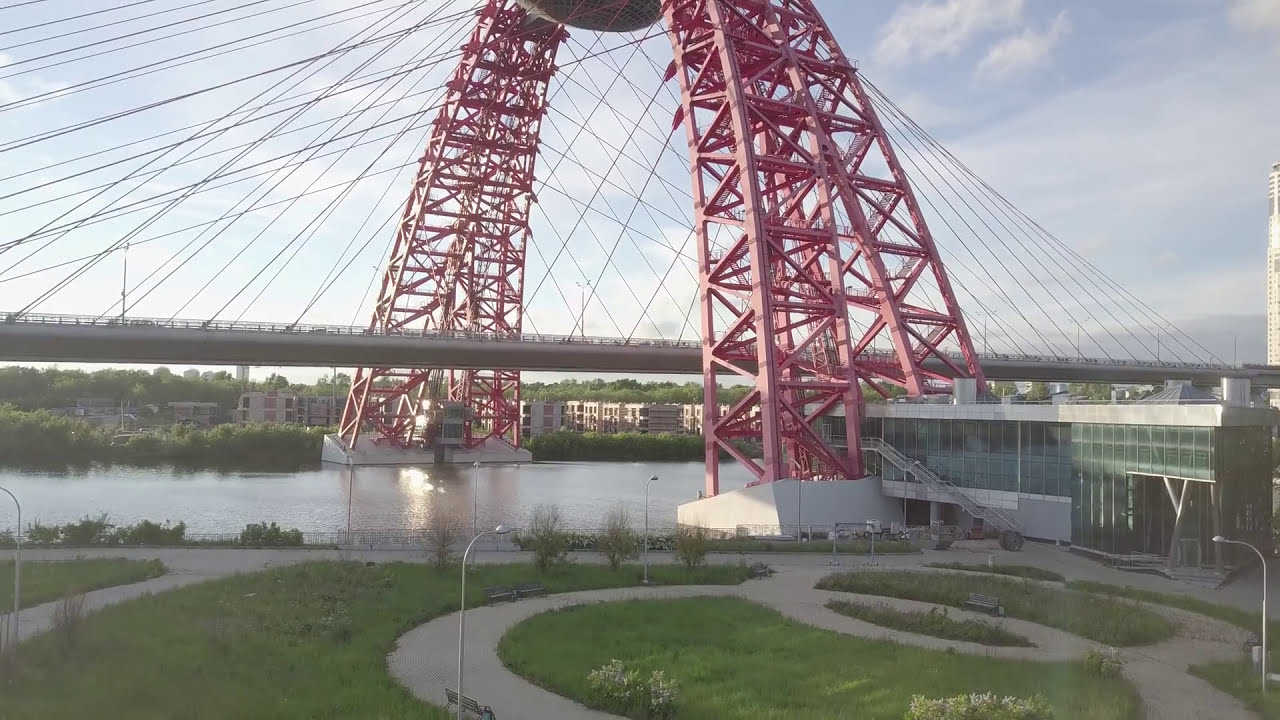The image depicts a large, concrete suspension bridge spanning a river, extending from the left to right of the frame. This architectural marvel is supported by a striking red arch structure, situated prominently in the center, which curves gracefully over the bridge. Numerous cables descend from the top of this arch, connecting to various points along the bridge, showcasing a feat of modern engineering.

Below the bridge, several buildings are visible. Notably, to the right of the arch, there's a multi-storied, predominantly glass building with green-tinted windows and no walls. Adjacent to it, and underneath the bridge, more buildings are scattered along both the left and right sides.

In the foreground, there is a serene park area with well-maintained grass and interconnected walking trails. The scene is dotted with streetlights that illuminate the pathways. The park is characterized by its small grassy islands that separate the walkways, creating an inviting and tranquil space.

The background of the image features an array of additional buildings and a picturesque sky, primarily blue with scattered white clouds, adding to the overall serenity and balance of this urban landscape.